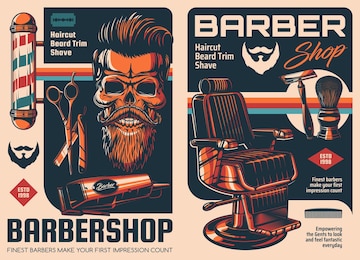This is a vibrant promotional image for a barbershop, set against an orangish-tan background with red, white, blue, and orange hues. Dominating the left side is a classic candy-striped barbershop pole enclosed in a glass cylinder with ornate orange metal finishes at both ends. Adjacent to the pole is a stylized skull with meticulously groomed hair, a beard, and a mustache, symbolizing the quality grooming services offered. Surrounding the skull are essential barber tools: a pair of scissors, a traditional straight razor, and an electric razor, encapsulating the full range of services available. The top-left corner features bold black text that reads “haircut, beard, trim, shave.” Beneath the skull, the phrase “Barbershop: Finest barbers make your first impression count” reinforces the shop’s commitment to excellence.

On the right side, another segment of text reads "Barber, Haircut, Beard, and Trim" accompanied by the silhouette of a beard with a mustache logo. Featured prominently are a lather kit with a standard razor, and a retro-style, orange barber chair complete with a side lever and footrest, evoking a sense of nostalgic craftsmanship. This rich assortment of classic barber imagery, paired with modern marketing elements, showcases the blend of tradition and contemporary style, making it an inviting and professional depiction of the barbershop experience.